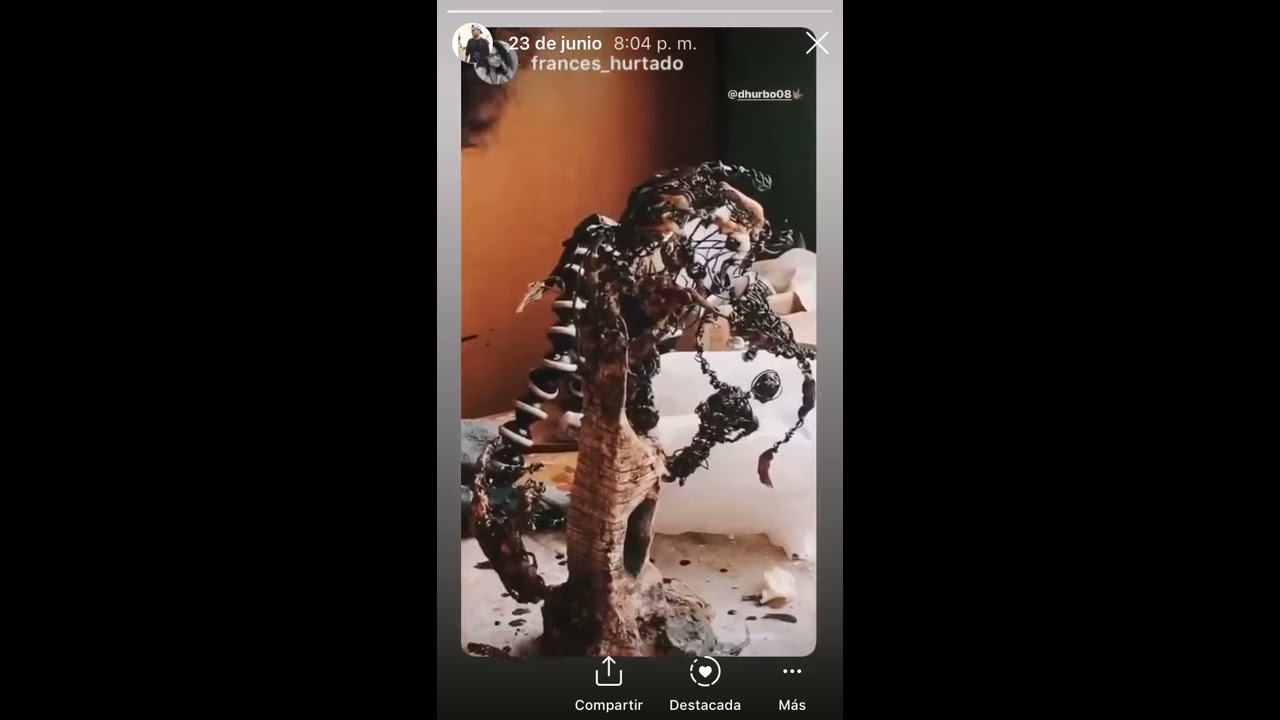This image is a horizontally rectangular screenshot from an Instagram story, primarily showcasing an abstract installation art or sculpture. The photograph is enclosed by wide black bands on either side, with the central focus in a narrower rectangle. The Instagram story was posted by the user 23Djunio at 8:04pm, and it’s a repost from Francis Hurtado. At the top, the screenshot shows profile pictures and usernames, while the bottom includes options to share or like the story.

The central image depicts a complex and intriguing structure, likely an artwork or sculpture made from a variety of materials. This structure appears to be constructed from metal objects, wires, and possibly components like a gorilla tripod - a circular, flexible tripod often used in photography. The sculpture's base is brown, and it extends upwards with black arms, wires, and other intricate elements, some of which dangle or protrude. On the left side of the sculpture, you can observe a series of circular forms that may represent a tail. The installation is set against a chocolate brown wall and placed on a light-colored surface, suggesting an indoor setting, possibly an artist's studio. The background also hints at some orange hues, adding to the overall complex visual presentation.